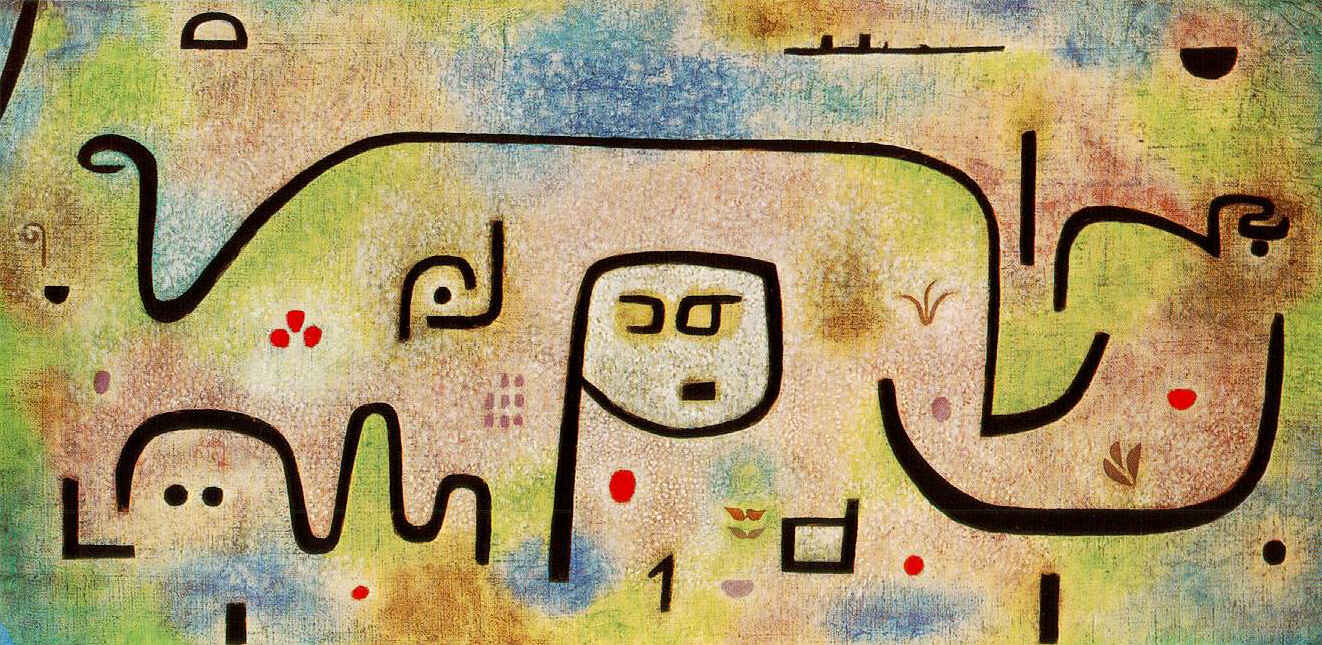The image is a detailed representation of Paul Klee's work titled "Insula Dulcamara," crafted in the 1930s as an example of abstract expressionism. The painting features a vibrant palette with pastel shades of blue, light green, and yellow, interspersed with light browns and bright red dots. The artwork is characterized by whimsical, black stylized line drawings that meander across the canvas, forming shapes open to individual interpretation. This piece includes elements that resemble eyes, faces, and even a ghost-like figure with wavy lines and eyes, adding to its enigmatic charm. The background presents a harmonious blend of pastel hues, against which the playful black lines stand out, creating a cheerful and engaging visual experience. The painting's clarity is precise, highlighting the intricate details and vivid colors without any text or signature visible. The lighting is bright and even, allowing each element of the art to be seen clearly. Overall, "Insula Dulcamara" by Paul Klee is a distinguished abstract expressionist piece that invites viewers to derive their own meanings, whether they see a cityscape, a bird, or purely abstract forms.